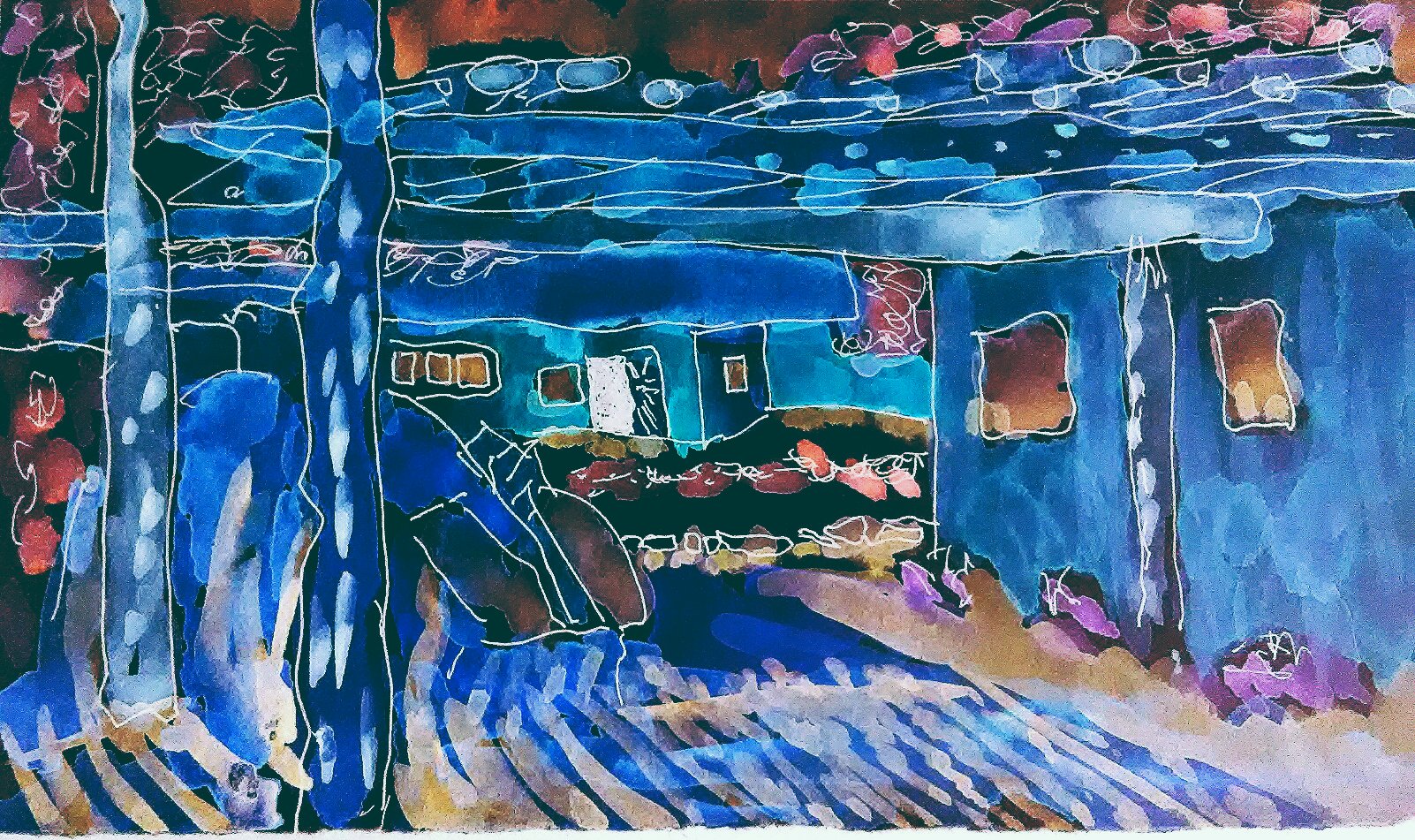In this intricate painting, the dominant hue is blue, creating a sense of depth and tranquility. The bottom portion showcases a blue floor adorned with delicate white and purplish lines. Just to the right, the color palette shifts to a combination of white and brown, interspersed with unique purple rock-like structures. Here, a blue building begins to emerge, accentuated by a central purple rod-like structure. Flanking this central feature are two squares, artistically shaded in hues of yellow and brown.

Above this architectural formation, a series of horizontal blue lines stretch across the canvas, interspersed with blue geometric shapes, adding layers of texture and dimension. To the left, two vertically aligned blue vines stand tall, juxtaposed against a collection of pink objects and a stark black background, creating a striking contrast. The same black background threaded with pink elements is also noticeable towards the top of the painting. The very top of the artwork gradually transitions into an orangish hue, adding a warm, glowing finish to the composition.